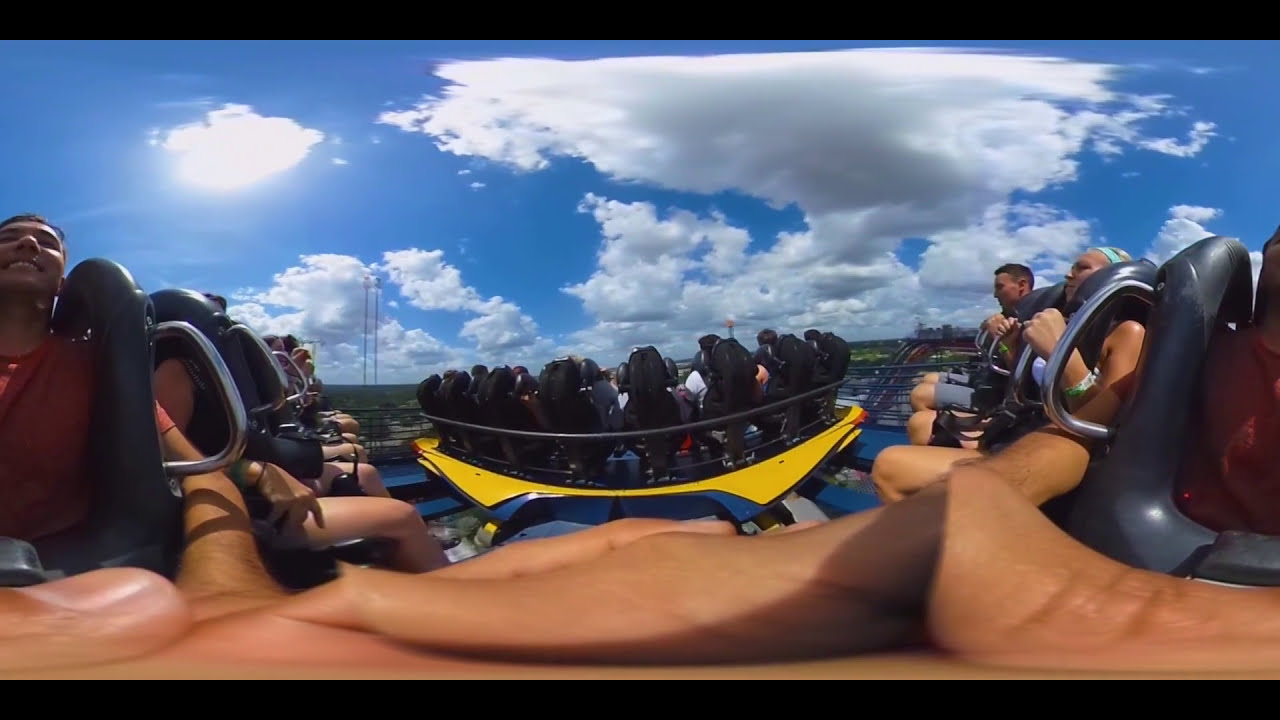The image captures a panoramic view of an intense roller coaster ride, possibly set in an amusement park like Cedar Point. High up on the track, two interconnected carts—painted yellow, blue, and red—are filled with riders who are securely fastened in black seats with silver over-the-shoulder restraints. The ride's blue metal structure contrasts with the vivid blue sky, which is dotted with puffy white clouds and a bright sun.

In this panoramic shot, the orientation is slightly distorted, causing some elements to appear warped. For instance, the riders on the left and right sides seem to be facing each other due to the photo splicing. You can identify a person on the left side with dark features, smiling broadly, showcasing his teeth and wearing a red shirt. His fingers, also distorted, appear knotted in the bottom foreground.

The central part of the image shows the backs of another row of tightly strapped-in riders. To the far left, you can see another intense drop of the coaster, while in the background toward the right, another group of people appears, lined up in their high-back chairs, ready for a thrilling experience. The overall setting is way up high, aligned with the clouds, emphasizing the ride's height and the vast, bright blue sky surrounding it. The atmosphere conveyed is one of excitement and fear as the riders brace for the adrenaline-pumping descent.